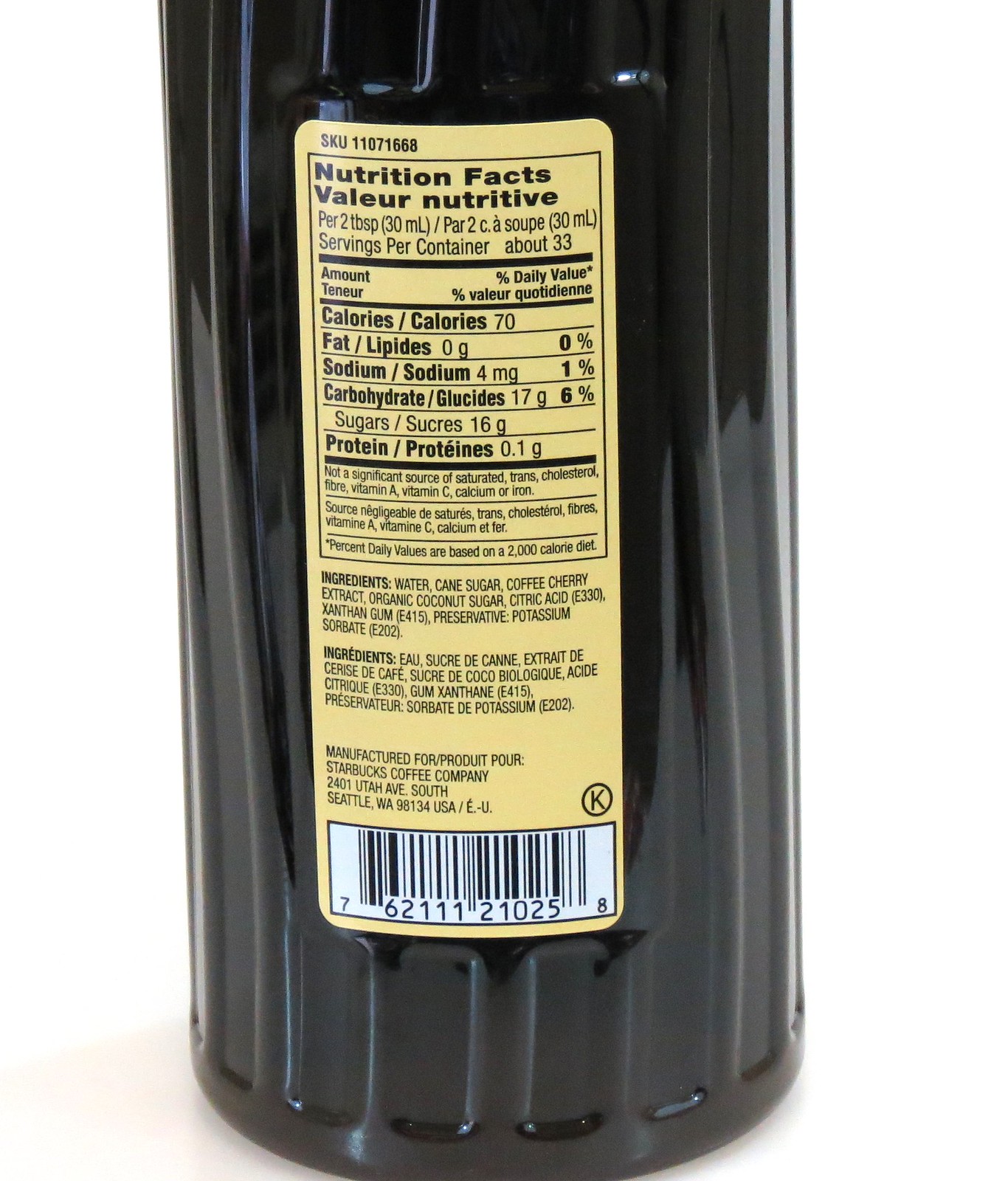A detailed close-up shot of the back of a clear plastic bottle containing a coffee beverage. The bottle features a nutrition facts label in a foreign language, possibly Portuguese or Italian. The label includes ingredients like water, cane sugar, and certified coffee extract. The bottle itself is transparent, allowing a glimpse of the dark brown coffee drink inside. The label is primarily yellow and also displays a black and white barcode. The overall color scheme of the image includes shades of brown and black from the coffee and yellow from the label, providing a stark contrast against the white text and barcode.